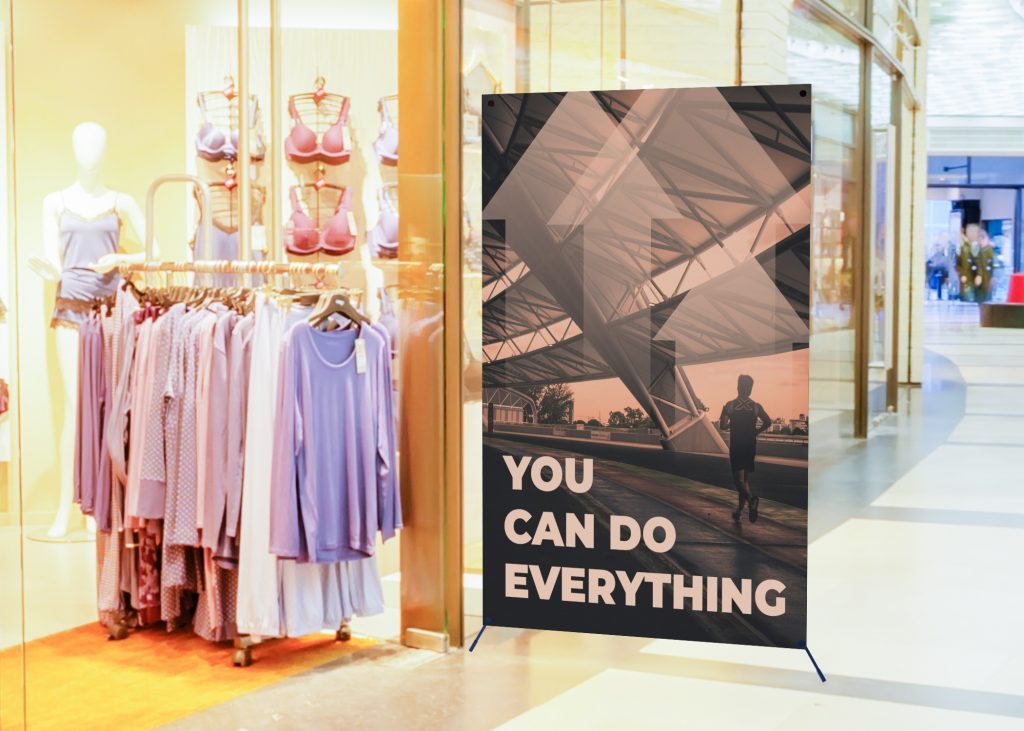The photograph depicts the entrance to a women's fashion store in a mall. On the left side of the image is an open storefront showcasing a rack filled with women's sleepwear, including long-sleeve tops, pants, and various clothing items in pink, blue, and white. In the background, against the wall, several racks display bras primarily in pink and blue. A white mannequin dressed in blue attire is also visible.

Prominently featured next to the store’s entrance is a life-size black-and-white poster of a man running, with the motivational slogan “You can do everything” at the bottom. The poster stands out as a key element of the scene. To the right of the store, a walkway leads to other stores in the mall, highlighting the setting as a shopping center. Overall, the image captures the vibrant and inviting entrance of the women's fashion store, accentuated by the motivational poster.